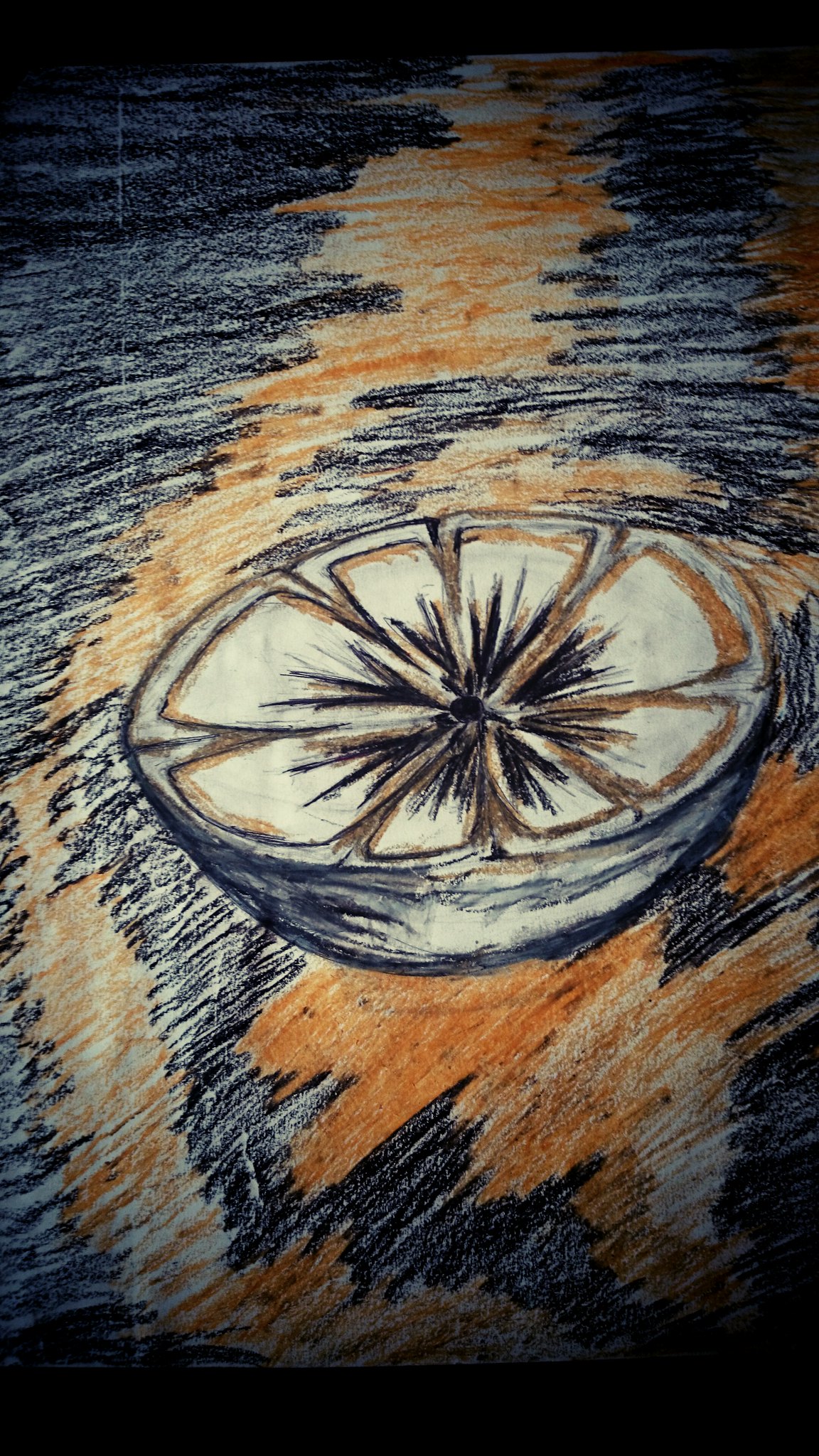The image depicts a detailed colored drawing, created using colored pencils or possibly crayons, on a white sheet of paper. The main focal point is a fruit that appears to be a half-sliced citrus, resembling an orange or a lemon, with its inner segments meticulously shaded. The inner sections of the fruit display shades of black and orange, giving it a striking, dimensional appearance. The fruit seems to be floating, with the background composed of swirling patterns of blue, orange, and black scribbles, adding a sense of motion and chaos. The top and bottom of the image are particularly dark, framed by intensive black shading, which enhances the vibrant contrast of the orange fruit against the dynamic, multicolored backdrop.